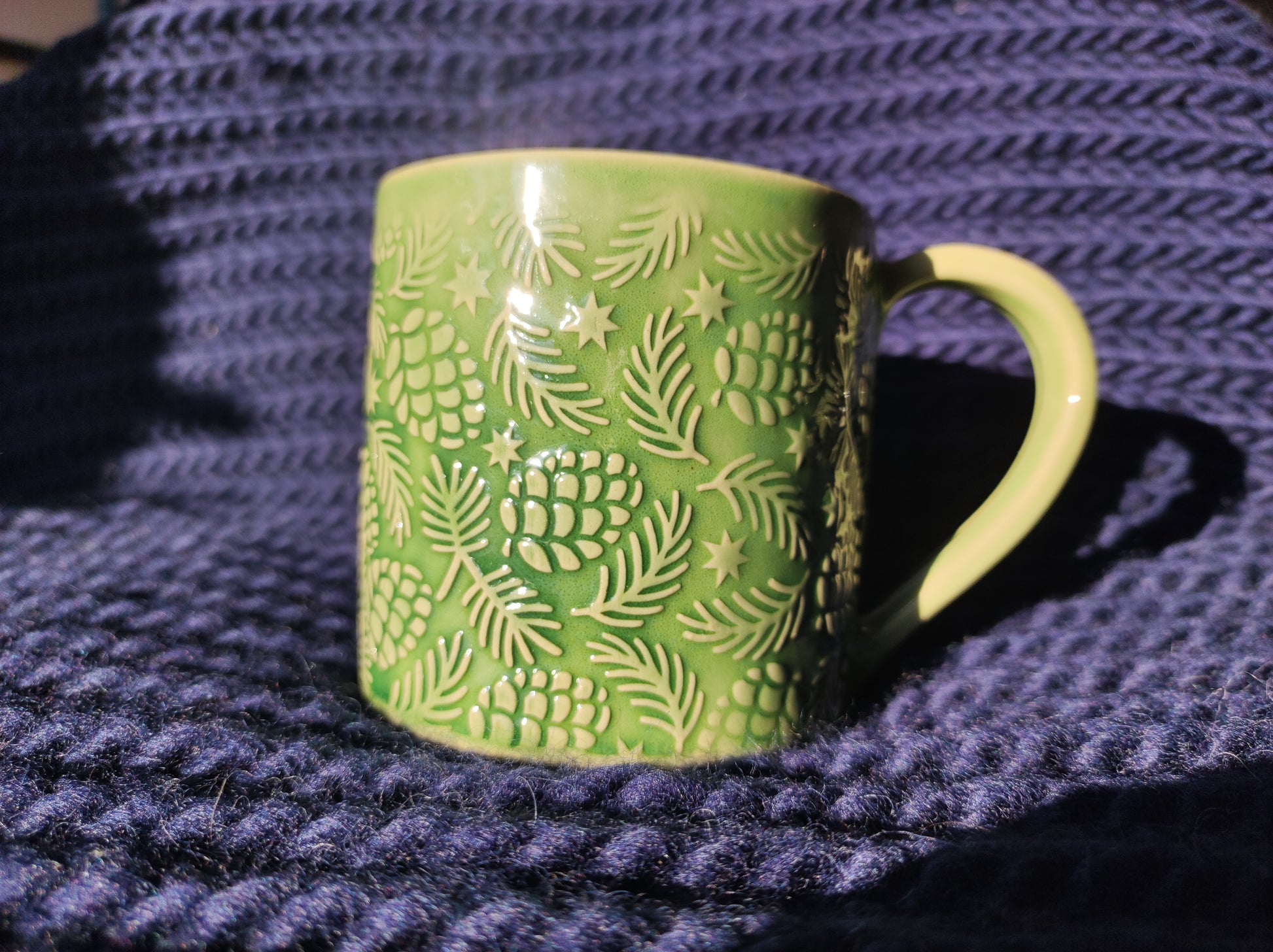This horizontal rectangular image is a detailed close-up of a green mug adorned with decorative pine branches, pine cones, and stars. The mug features a light green, yellowish handle positioned on the right side, with matching yellow accents within the designs. The center of the front of the mug prominently showcases a pine cone, surrounded by leaves and stars, with this pattern repeating around the mug. The mug is resting on a richly textured, rope-like blue placemat, which could also resemble a homemade knitted blanket. The vibrant blue material contrasts with the dark background visible in the lower left corner. Both the mug and its handle cast discernible shadows on the blue textured surface, adding depth to the composition. The overall image is highlighted by the intricate details and the harmonious play of colors and textures.